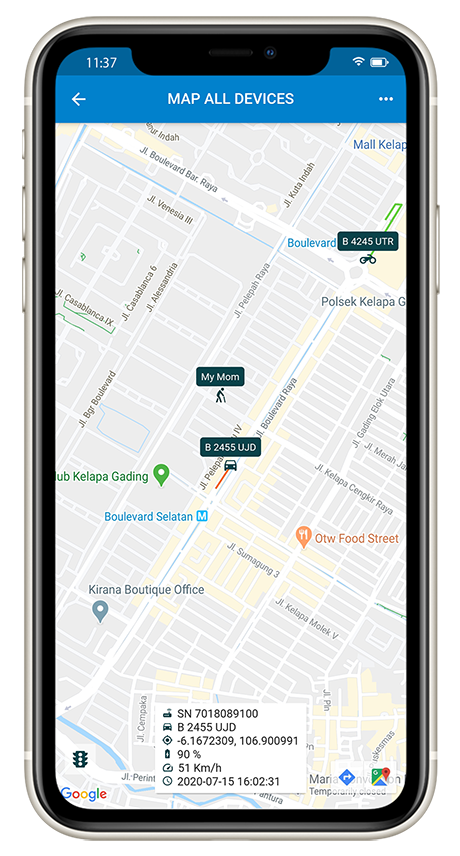A screenshot of a mobile phone displaying a detailed digital map interface. The phone shows a time of 11:37, with a strong signal and a nearly full battery at 90%. The screen features a blue-themed interface, highlighted by a blue background with a left-pointing arrow and the text "Map All Devices" centrally positioned, along with three horizontal dots on the upper right corner.

The map itself identifies several key locations and devices. It marks the presence of "my mom," "B4245UTR," and "B2455UD" at different points. Notable landmarks include "OTW Food Street," a restaurant, "Karina's Boutique Office," and "Club Kelepa Gatting." The phone's screenshot captures all these details against a predominantly white background.

Additionally, the date displayed is July 15, 2020. The phone is enclosed in a clear case, allowing the black rim of the device to be visible.